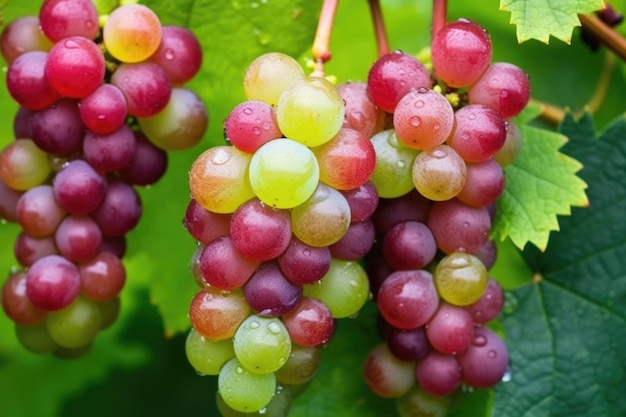The image is a photorealistic close-up of three clusters of grapes hanging from vines against a backdrop of green leaves. The central cluster and the one just to its right are primarily composed of purple and green grapes, with the rightmost cluster displaying a mix of purple, red, and some green grapes. The leftmost bunch, slightly larger and to the left side of the image, features predominantly red and green grapes. Water droplets are visible on the grapes, enhancing their freshness and making them look ripe and ready to eat. The background leaves, with varying shades of green from bright lime to dark tones, are out of focus, which draws attention to the detailed and textured grapes. There is no text in the background, and the perspective of the image is straight on, emphasizing the lush and inviting quality of the grapes.